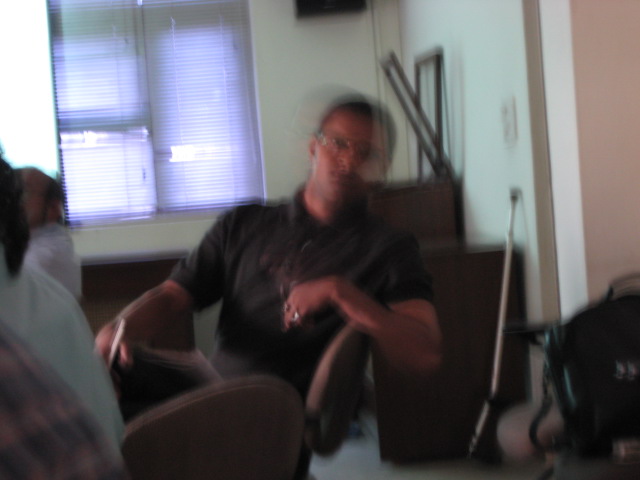The image is a blurry photograph taken indoors, depicting a Caucasian man wearing glasses and a black t-shirt, possibly a button-up shirt, seated in a brown rolling chair. The man, who is facing the camera, appears to be leaning slightly backward in the chair. He has his right arm extended in front of him, possibly resting on what seems to be a table, while his other arm rests on the back of the chair. The room features a white wall with two windows partially covered by blinds and there is a noticeable double-image effect around the man's head, giving the impression of motion. Behind the man, slightly to the right, a pole lies against the wall. Additionally, the scene includes indistinct equipment in the right corner, a small brown box in the top corner, and two picture frames leaning against the wall. The presence of two other individuals in white shirts can be observed, sitting with their backs to the camera.